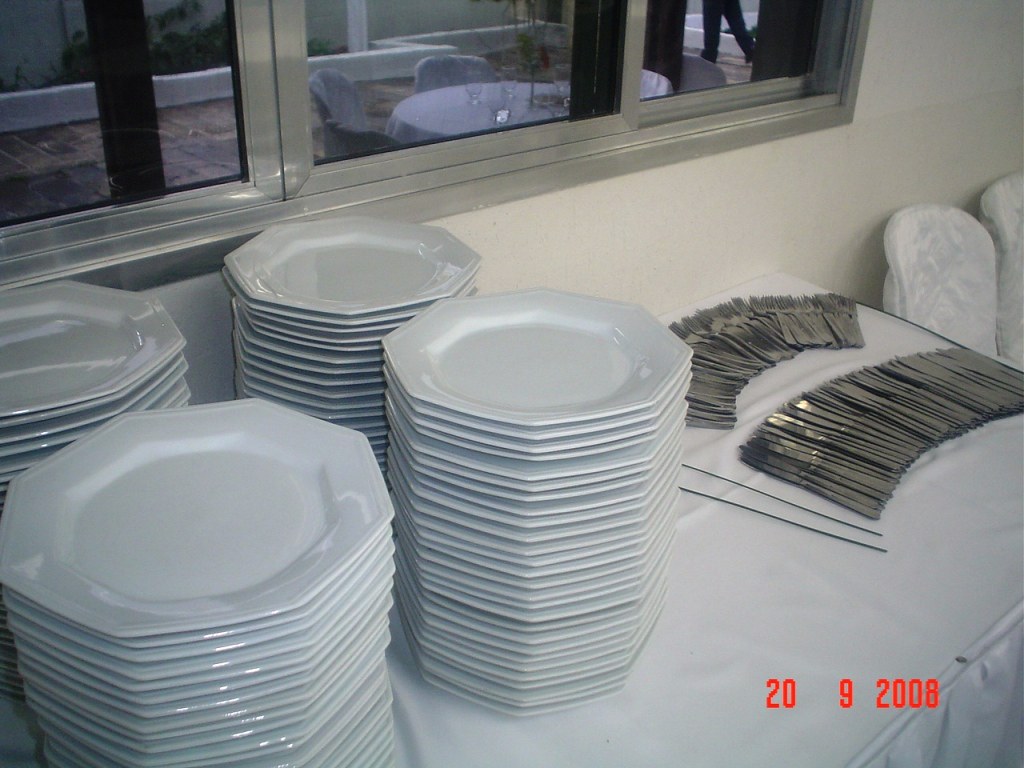The image, dated September 20, 2008, in red text at the bottom right, captures a well-organized display of dinnerware on a white table covered with a white cloth. The table is set indoors, possibly at a formal event or wedding buffet. At the forefront, there are four neat stacks of pristine white, octagonal plates arranged in two rows. To the far right of the plates, a long line of polished knives is neatly aligned, with a stack of gleaming forks positioned just behind them. Beyond the table, the scene extends to a window that reflects an outdoor setup with chairs and glasses, suggesting a continuation of the event's dining area. The overall ambiance hints at the onset of evening as it's getting dark outside. Additionally, on the right side of the image, partially visible are the walking legs of a person, further adding to the lively atmosphere of the gathering.